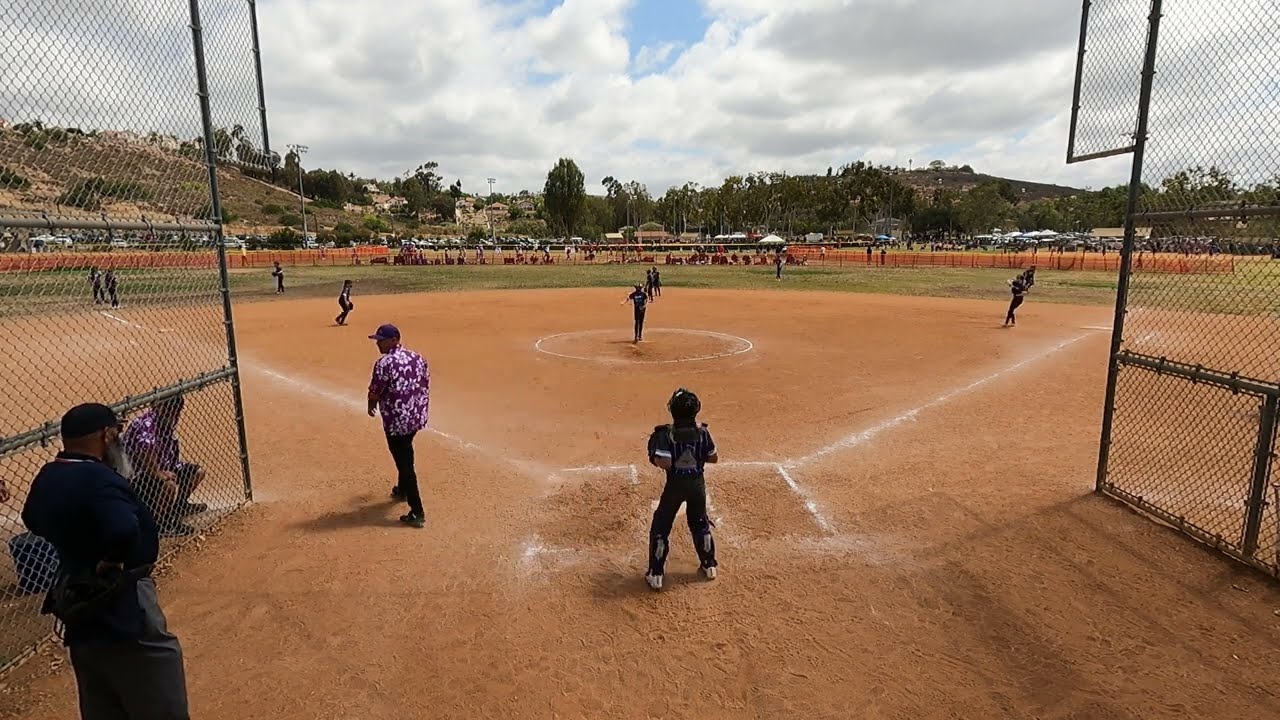The image captures a lively baseball game in progress on a predominantly tan, sandy dirt field, marked with white chalk lines defining the bases and pitcher's mound. Central to the image is a young catcher wearing white tennis shoes, black pants, a black jersey, and black protective gear, stationed amidst a chain-link fence backdrop of tall batter's cages on either side. In the bottom left corner, a referee outfitted in black padding, a black baseball cap, polo, and pants is visible. The scene includes a pitcher and several young players scattered around the field, a stark contrast to the adults present. The distant background reveals a blue sky dotted with clouds, lush greenery, and additional field space, though the dominant hues remain the brown of the dirt and the white of the chalk lines.